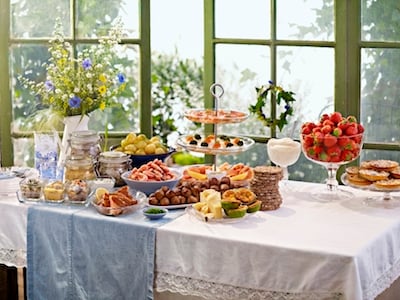The image showcases a beautifully arranged long trestle table set for tea, laden with a variety of delectable treats. Dominating the display is a large glass bowl with an elegant stem, brimming with ripe, red strawberries. Several cake stands are placed strategically across the table, laden with an assortment of pastries and small cakes, including a prominent three-tiered stand showcasing an array of little cakes and delicate pastries. Smaller glass dishes in the foreground hold an assortment of bite-sized treats, likely including savory options such as sausage rolls and pigs in blankets, though the exact contents are not clearly discernible. Adding to the aesthetic appeal is a tall white jug adorned with flowers, bringing a touch of elegance to the table. The entire setting is enhanced by white tablecloths, two of which feature intricate lace edgings, adding a classic, refined touch to the lavish spread.